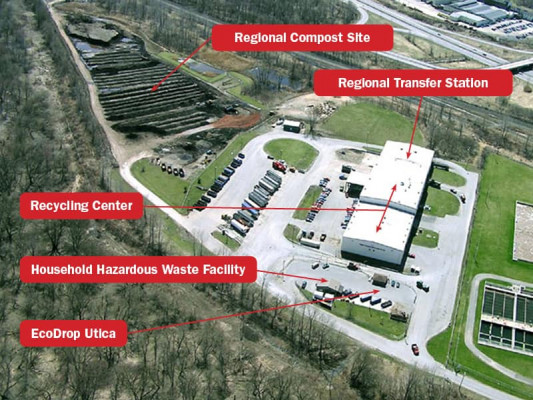This aerial color photo captures a sprawling recycling facility, prominently situated within an open field. At its core lies a white building, surrounded by a network of paved roads and lush green grass. The image is annotated with red rectangles and white lettering, clearly labeling various key areas of the facility. These labels point to the regional compost site, regional transfer station, recycling center, household hazardous waste facility, and EcoDrop Utica. The compost site and plant appear extensive, likely aimed at promoting soil enrichment and supporting plant growth. The entire setup underscores the facility's commitment to reusing materials and aiding the economy. The photo provides a comprehensive overhead view, highlighting the intricate layout and diverse functionalities of this industrial area.